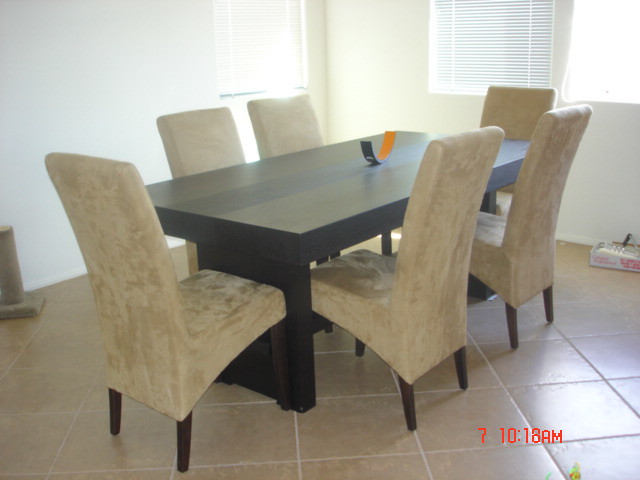This color photograph captures a sunlit dining room from an interior perspective, taken at 10:18 a.m., as indicated by the red print in the bottom right corner. The focal point is a robust, dark brown rectangular wooden table, positioned diagonally and supported by a wide leg that spans its full width down to the floor. Surrounding the table are six high-backed, armless chairs, upholstered in plush, velvety beige fabric, creating a harmonious contrast with their dark wooden legs, which are short at the back and taller at the front, adding a distinct artistic touch while maintaining functional integrity.

In the center of the table sits a striking U-shaped decorative object, boasting a black exterior and an orange interior, serving as a noteworthy centerpiece. The floor is tiled with large beige tiles arranged in a diamond pattern, complemented by the room's white or green walls, although the exact hue is ambiguous. 

Three windows adorned with white Venetian blinds permit the morning sunlight to gently filter into the room, illuminating the scene subtly. Among the furnishings, a white box with pink indecipherable writing is positioned on the floor beneath one window, while a grey object, partially visible, sits off to the left side of the photograph. Notably, a cat scratch tower is also present near the table, adding a homely touch to the meticulously arranged space.